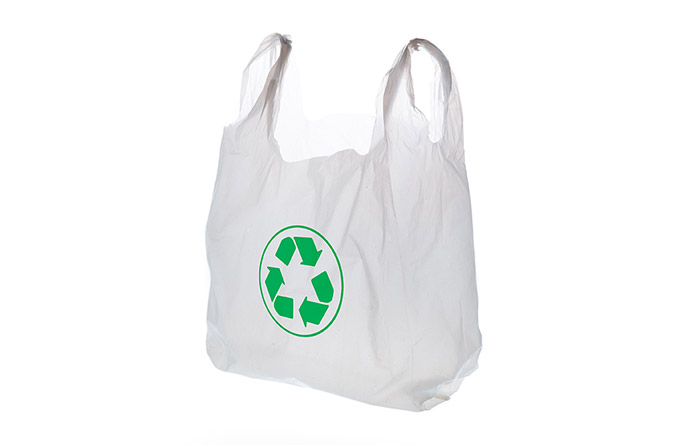The photograph showcases a simple, white plastic shopping bag standing against a plain white background. The bag, made of thin, semi-translucent plastic, has its handles pulled up and fully extended. Although the bag appears full, its contents are not visible. Prominently displayed in the center of the bag is a green recycling logo, consisting of a circle with three green arrows folded over and pointing at each other to form a continuous triangular loop. The minimalist composition emphasizes the solitary bag and its prominent environmental symbol.